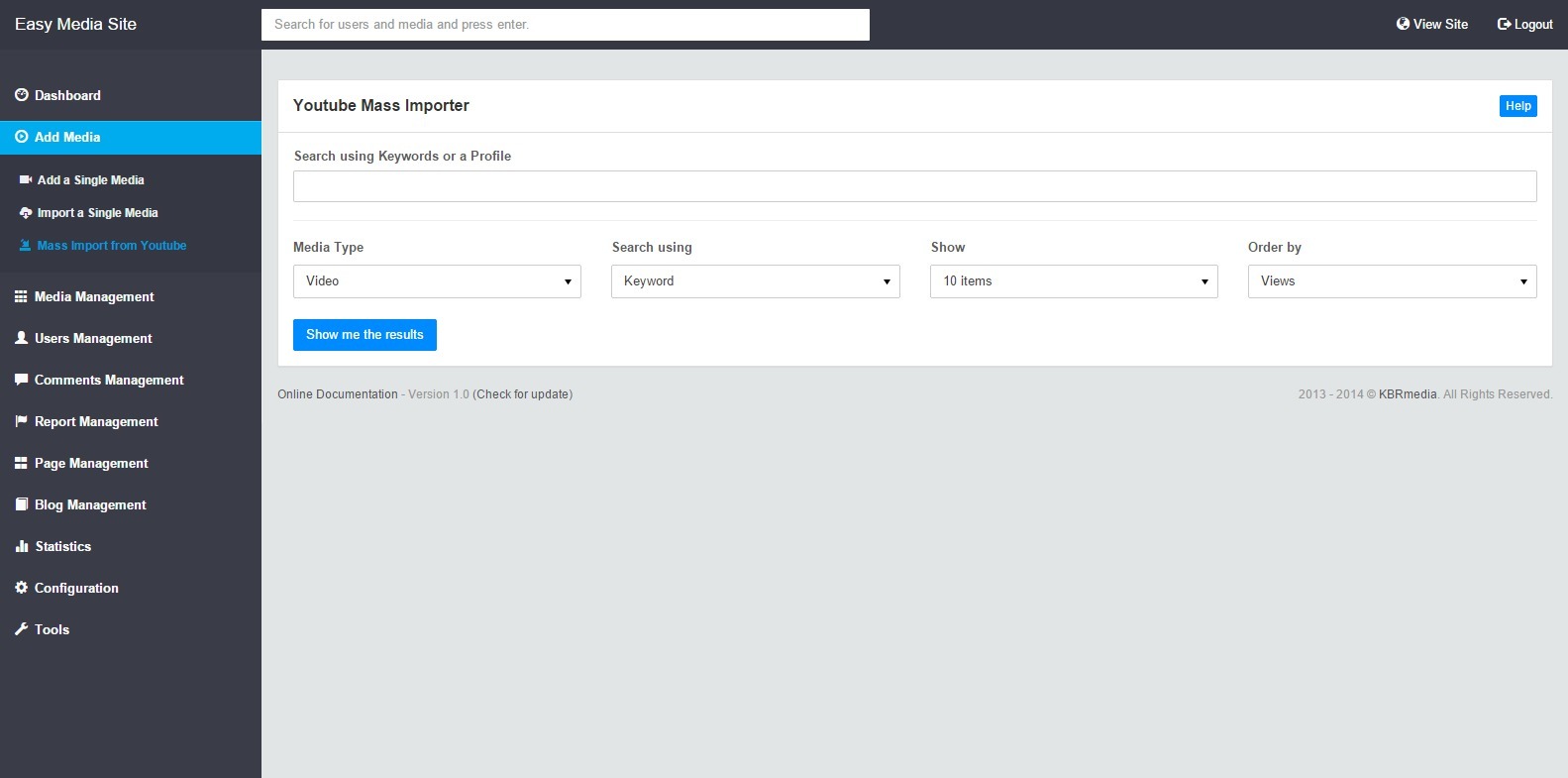The image depicts a user interface of a website called "Easy Media Site." At the top of the screen, a grey banner spans horizontally. On the top left of the banner, "Easy Media Site" is displayed in white text. To the right of this label is a long white search bar. Further right, the banner includes a "View Site" link and a "Log Out" button.

Continuing down the left-hand side of the screen, the grey banner extends into a series of large, wide panels with various selectable headings. The currently selected heading is "Add Media." Other options visible in this panel include "Dashboard," "Add a Single Media," "User Management," "Media Management," "Comments Management," "Report Management," "Page Management," "Blog Management," and more, including tools for configuration.

On the right-hand side of the screen, there is a large grey window that occupies the majority of the page. Inside this window, approximately half the space is taken up by a white rectangle. At the top of the white rectangle, the black heading reads "YouTube Mass Importer." Below this, there is a long input field designated for entering search criteria, such as keywords or a profile. Several pull-down menus are arranged underneath; these menus allow the user to select options under "Media Type," "Search Using," "Show," and "Order By." At the bottom left within this white panel, there is a blue button labeled "Show Me The Results."